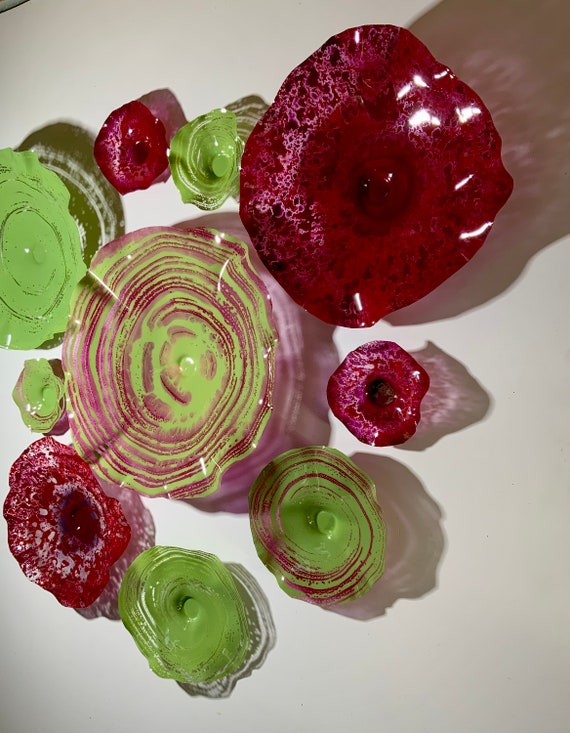The photograph showcases a top-down view of an arrangement of ten artistic glass plates, varying in size from relatively large to small, displayed at a glass-blowing exhibition. Each plate, intricately designed with a blend of red and green shades, exhibits a glossy and sometimes translucent appearance with light illuminating from the left side. The edges of these plates mimic the petal-like structure of flowers, enhancing their delicate and artistic nature. Central to the image, we observe a prominent pink and green spherical object, about the size of a 45 RPM record, displaying intricate wrinkles and standing out as a centerpiece. Surrounding this central piece, from top right and moving counterclockwise, the description mentions a green and white spherical object, a mauve-pinkish circular plate with white delineations, a green plate with transparent streaks, another glossy spherical object blending green with pink stripes similar to the centerpiece, a larger red and pinkish-mauve circular plate, a green circular object with clear patterns, a larger green and pink circular plate, a smaller red and white delineated spherical object, and finally, a large pink spherical plate with marble-like white streaks. Each piece is presented with its outer surface lying flat, emphasizing the vibrant and swirling interior designs.